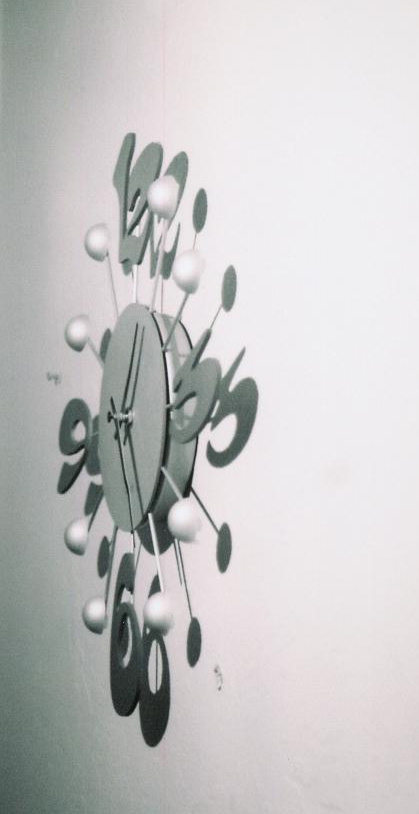A round clock hanging on a white wall is prominently featured in the center of the image. The clock face displays the numbers 12, 3, 6, and 9, with two small white dots situated in between each set of these numerals. Shadows can be seen behind each number, indicating a play of light and depth. The photo is presented in black and white, adding a classic and timeless touch. To the left of the clock, a small thumbtack can be seen embedded in the wall, contributing to the everyday realism of the scene.